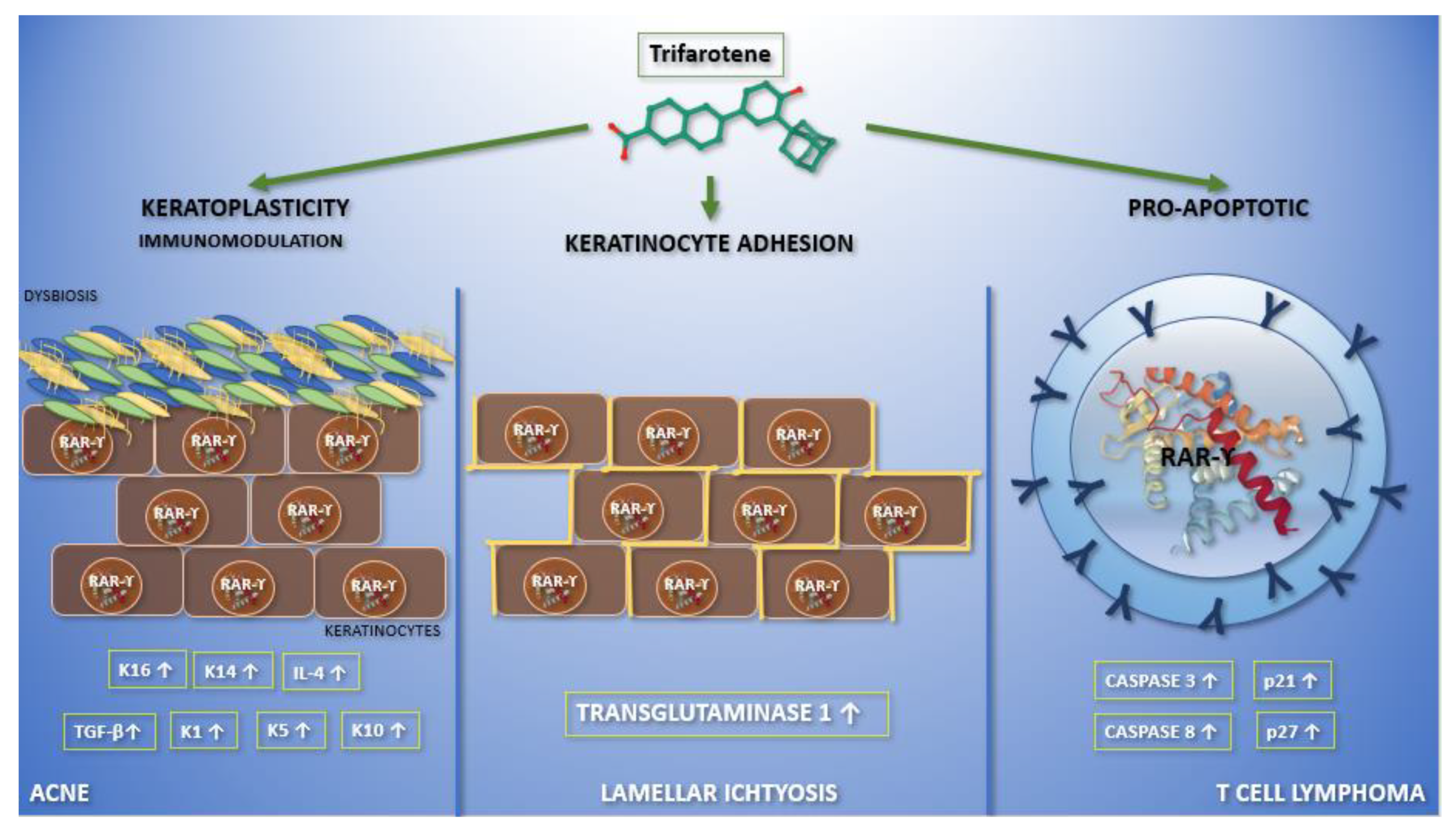The image is a detailed rectangular diagram, measuring about 5 inches wide by 3 inches high, with a blue background that fades to white at the top center. At the top center, there is a light gray outlined rectangle containing bold black text that spells out "Trifarotene." Below this, the chemical composition is depicted with hexagrams and red dots, flanked by three green arrows pointing left, down, and right. 

To the left, the left-pointing arrow is labeled with "Keratoplasticity" and "Immunomodulation" in black print. Below these labels, additional text reads "Dysbiosis" over illustrations of blue, green, and yellow ovals, followed by brown rectangles with circles inside them. Underneath, it states "Keratinocytes," and in the lower left corner, small rectangles with white print and arrows pointing up are labeled "Acne."

In the middle, the downward arrow is labeled with "Keratinocyte Adhesion," and the same brown rectangles appear again with "Transglutaminase" below them. A text that says "Lamellar Ichthyosis" appears at the very bottom.

To the right, the right-pointing arrow is labeled "Proapoptotic," leading to two circles. Inside the central circle, "R-A-R-Y" is printed, surrounded by different colored ribbons and smaller circles outside with the letter "Y." At the very bottom, "T-Cell Lymphoma" is noted.

The diagram is essentially divided into three informative sections, each representing different scientific and medical details: from keratoplasticity and immunomodulation to keratinocyte adhesion, to proapoptotic processes, all detailed with vivid colored diagrams and corresponding texts.